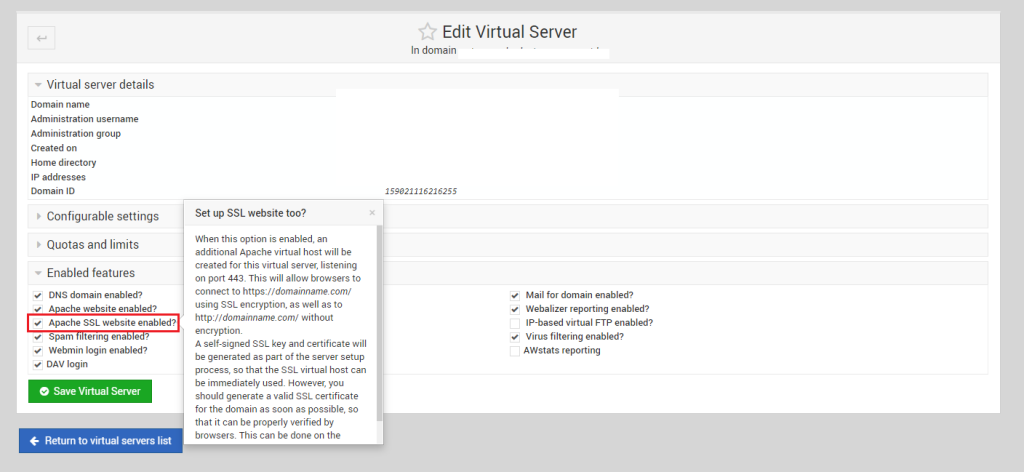In the image, there is a light gray background with a white central area displaying a web interface related to server management. At the top-left corner, there is a back arrow icon. Below it, the heading reads "Virtual Server Details" followed by a list of details including "Domain Name," "Administration Username," "Administration Group," "Created On," "Home Directory," "IP Address," and "Domain ID." 

Additionally, a menu is visible with options titled "Configurable Settings," "Quotas and Limits," and "Enable Features." The "Enable Features" section is expanded, revealing six checkmarked features, one of which is outlined in red and labeled "Apache SSL Website Enabled."

A green button labeled "Save Virtual Settings" is positioned beneath this list. A pop-up window overlays part of the screen, with the header "Set up SSL Website?" It mentions that when this option is enabled, an additional Apache virtual host for this server will be created and will listen on port 443. The pop-up includes two short paragraphs containing technical explanations.

Outside the white area of the interface, there is a blue button labeled "Return to Virtual Servers." On the far right of the pop-up, there are three checkboxes with inquiries next to them: "Mail for Domain Enabled?" "Mobilizer Reporting Enabled?" and "Virus Filtering Enabled?"

This image captures the process of setting up and configuring a virtual server.